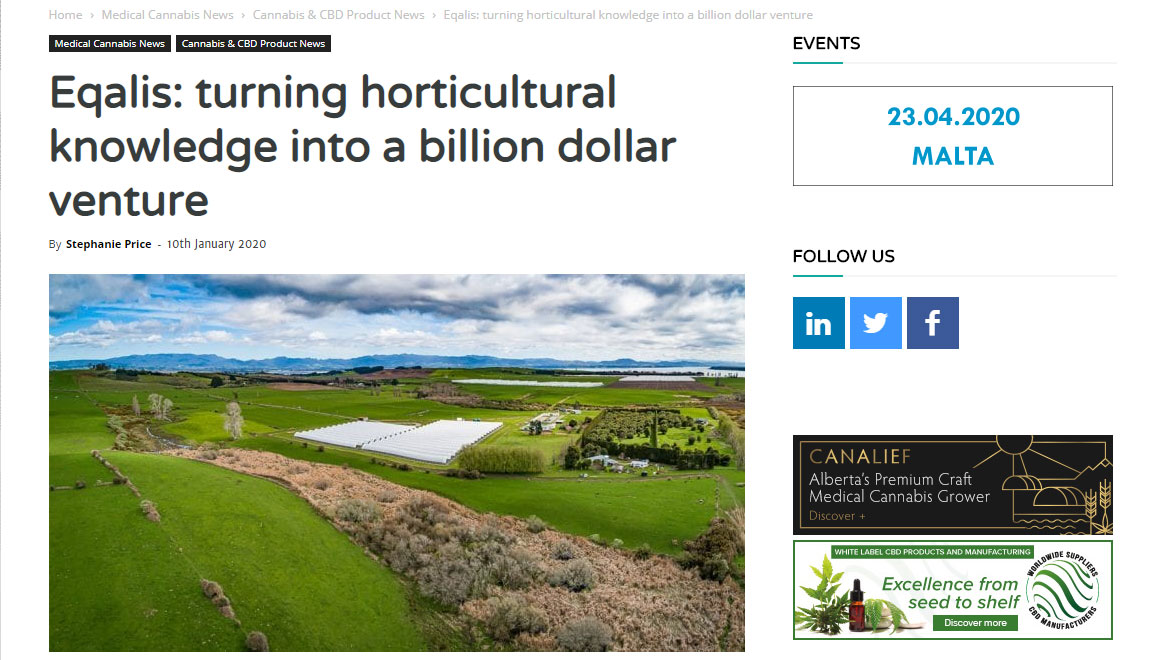Caption:
"An image captures a detailed article that appears to be suitable for both online publication and newspaper print, titled 'Equalis: Turning Horticulture Knowledge into a Billion-Dollar Venture' by Stephanie Price, published on January 10th, 2020. The photo showcases a vast grassy field area extending into the background. White rows of plants are visible, set against rolling hills or mountains in the distant backdrop. The sky above is a mixture of white and gray clouds, with patches of blue peeking through. To the right side of the image, an 'Events' section is highlighted, followed by a box stating '23-04-2020' and 'Malta', along with icons for LinkedIn, Twitter, and Facebook suggesting social media follow options. The bottom right corner features an advertisement for a cannabis grower, reminiscent of an olive oil label."